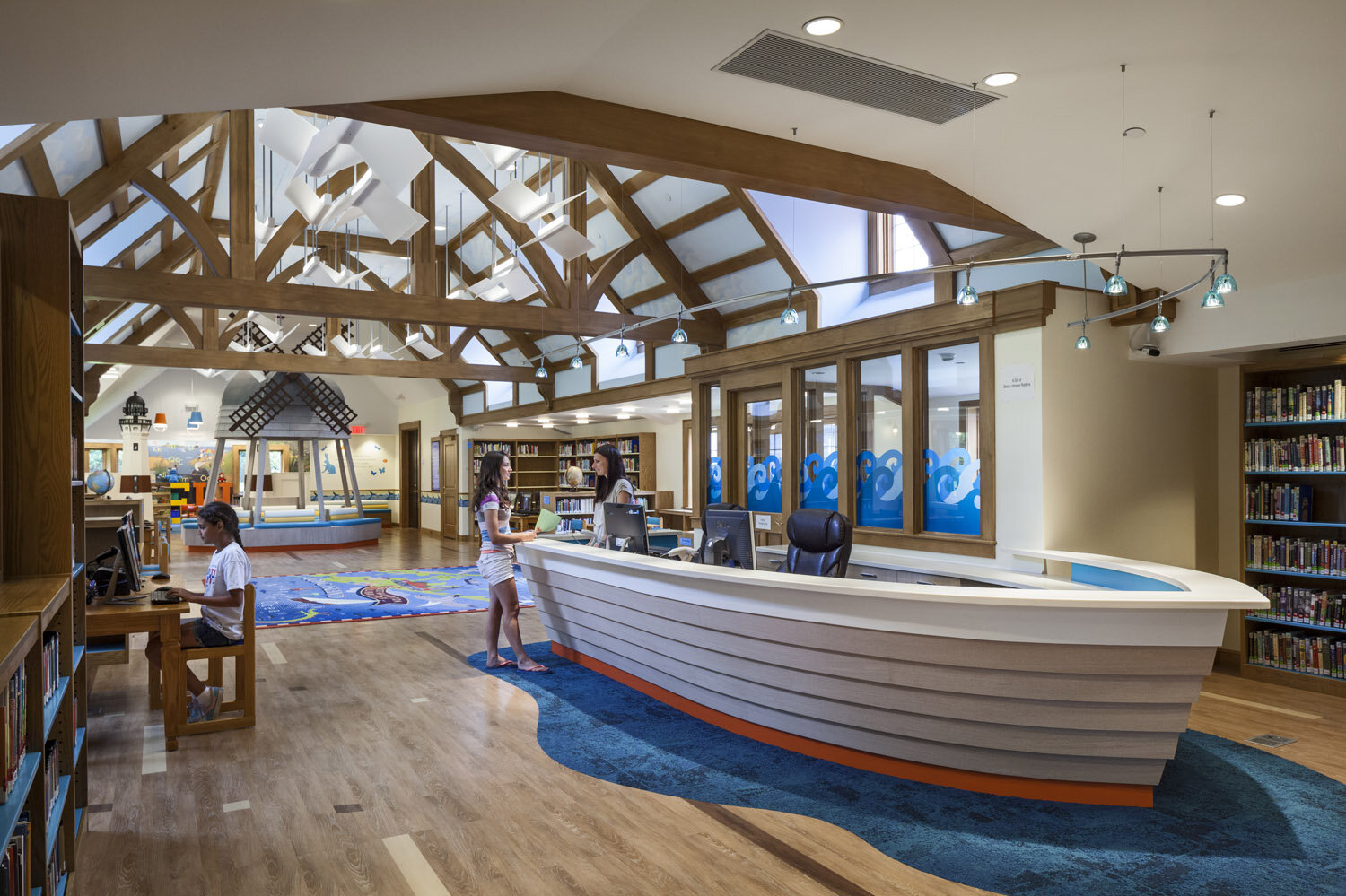The interior of the children's library in East Hampton is depicted in a detailed, colorful photograph. The library features a unique and captivating centerpiece: a boat-shaped desk adorned with a white rail and beige siding, accented by a red line at the waterline. This boat structure rests on a wavy blue carpet, giving the impression of sailing on a sea amidst the hardwood floor. The library is bathed in natural light streaming through the large A-frame roof with glass panels.

At the stern of the boat, two women with black hair engage in conversation. One wears flip-flops, short white shorts, and a striped t-shirt while holding a book, suggesting she might be a patron. The other woman, possibly a librarian, stands nearby. Surrounding them are shelves filled with books, each marked with small white stickers indicating call numbers.

A young girl, approximately 13 or 14, is focused on a computer at a desk on the left side of the room. Nearby, a globe and a windmill structure with four black blades add an element of whimsy, hinting at a playful, child-friendly environment. This richly detailed scene combines elements of practicality and imaginative design, creating an inviting atmosphere for young readers.

In the background, additional bookshelves and windows painted with blue ocean waves enhance the maritime theme. The right side of the room near the bow of the boat showcases more books, making the library not just a place of learning, but also one of visual delight and creativity.